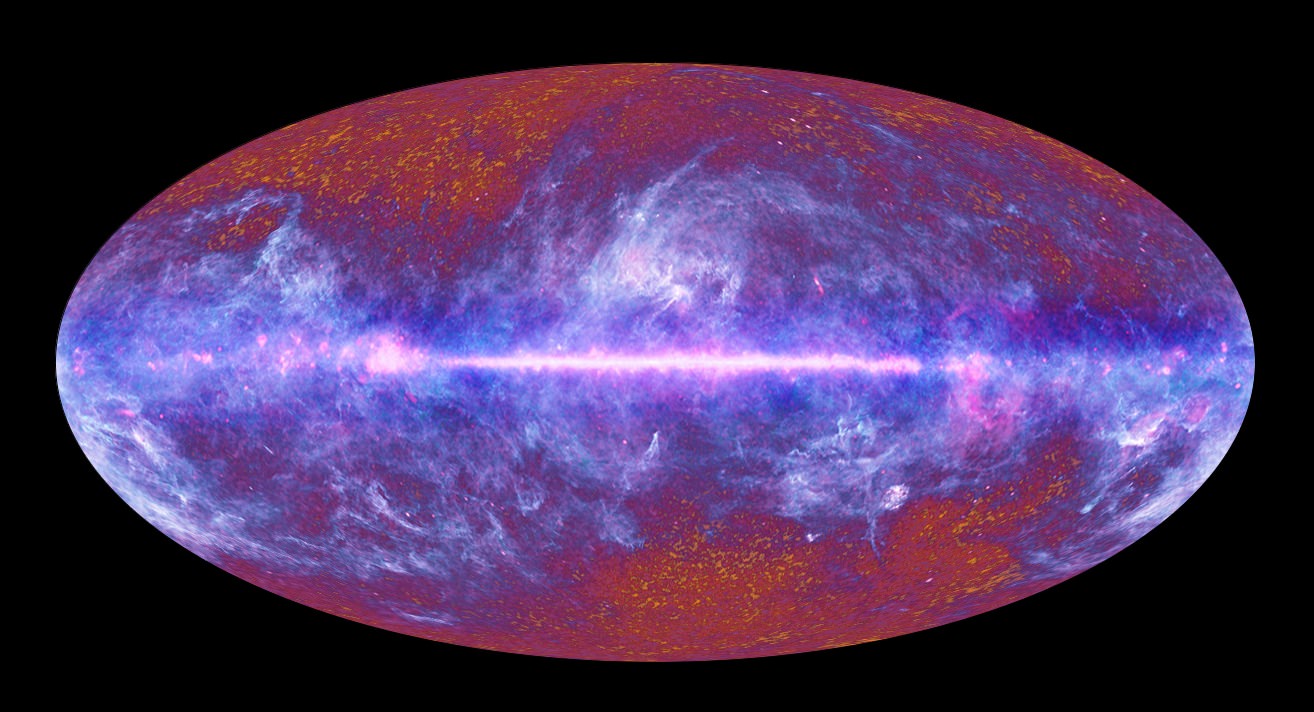This image features an oval-shaped representation of the known universe set against a solid black background. The universe is depicted with a variety of colors: the bottom and top display orange and brown hues, while the middle section is predominately blue with touches of purple. Speckled throughout are red, pink, and white, adding a densely clouded texture that makes it difficult to discern stars or constellations. A bright, beaming light, composed of pink and white, runs horizontally through the center, almost splitting the oval in half. This vibrant stroke of light is a prominent feature, drawing the eye across the elliptical shape, which spans from left to right like a cosmic equator. The overall impression is one of a vividly colored, AI-generated celestial map, blending abstract artistry with astronomical elements.